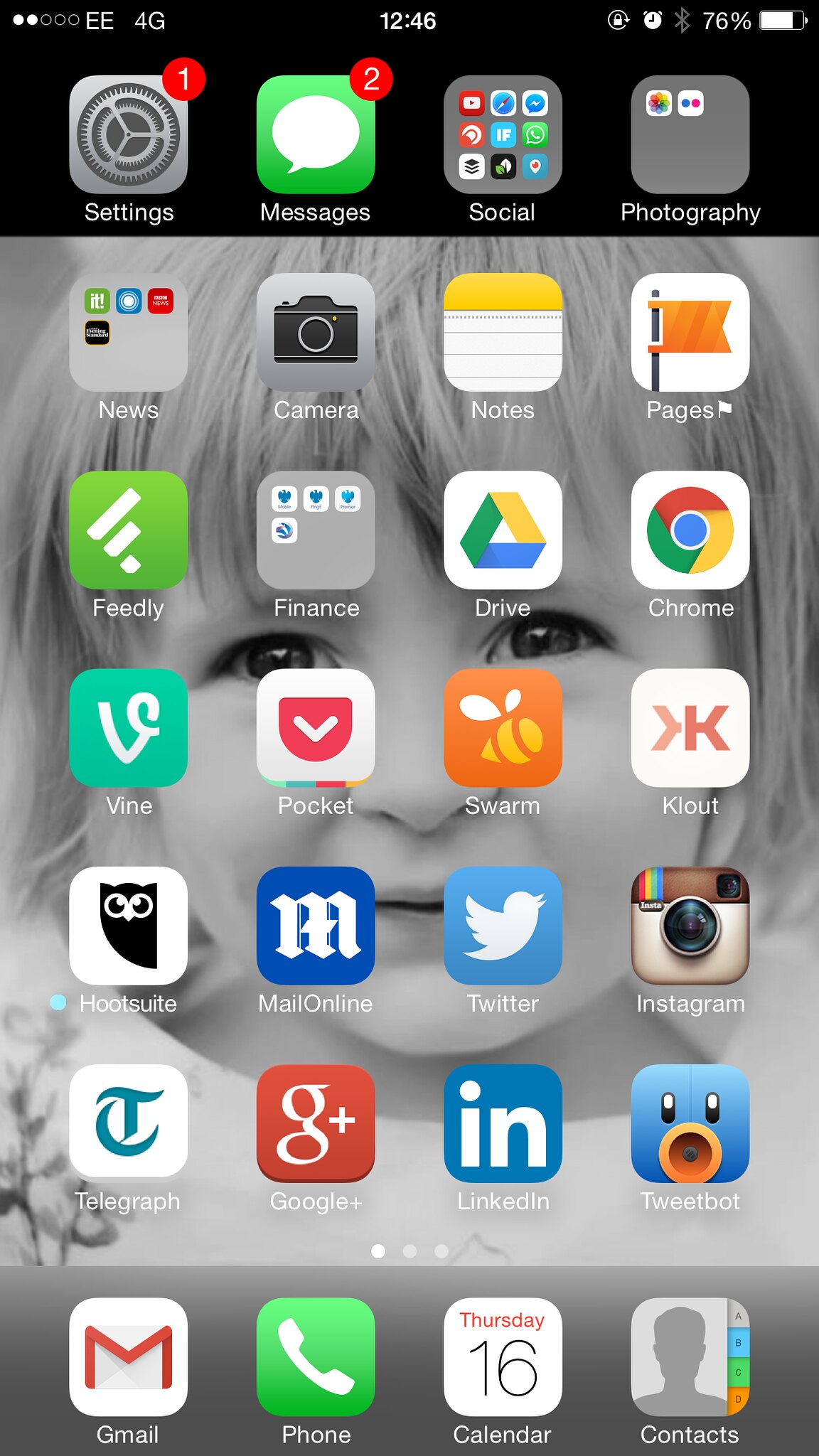This is a color photograph depicting the home screen of a smartphone. The screen features various app icons arranged in a grid. At the top of the screen, a black strip is present, displaying icons for settings, messages, social media, and photography, each represented by distinct logos. In the center of the top bar, the current time is displayed, while the battery indicator and network status (EE 4G) are positioned on the right and left sides, respectively.

The main section of the screen contains a grid of 20 app icons arranged in 5 rows and 4 columns. These icons include popular apps such as Twitter, Google+, Vine, Drive, and Pages. The background of the home screen is set to a black and white photograph of a baby, whose eyes are gazing directly at the viewer from the center of the screen.

At the bottom of the screen, a medium gray strip runs horizontally, featuring four primary icons: Gmail, phone, calendar, and contacts. The battery indicator suggests the phone has approximately 40% power remaining, as indicated by the two out of five dots. The overall composition creates a functional and personalized interface on the smartphone.